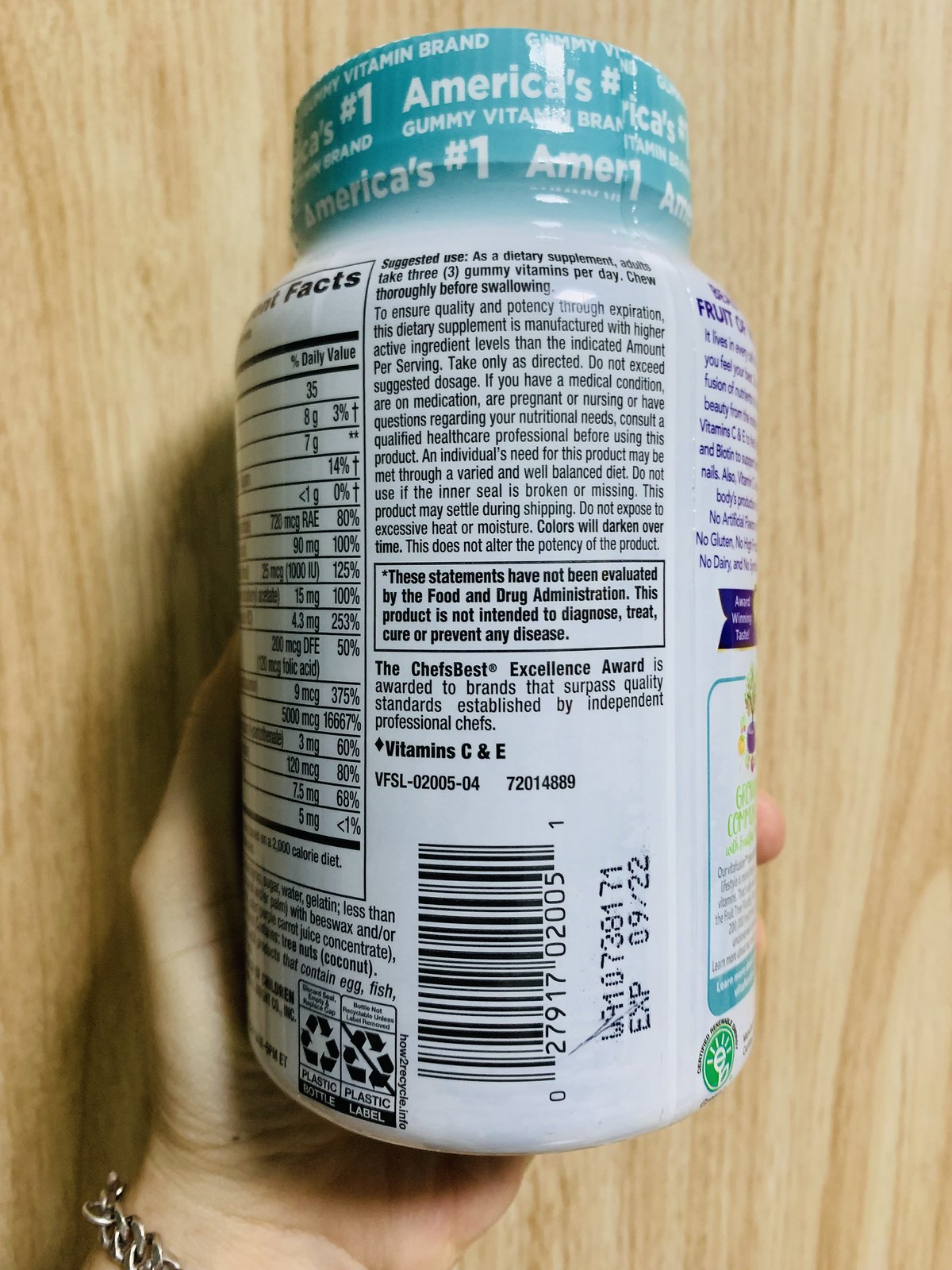In the image, a left hand is holding an unopened vitamin bottle with a prominent blue plastic cap featuring the text "America's number one gummy vitamin brand." Only the thumb and a couple of finger tips are visible, with the hand sporting a chain bracelet partially in view. The background consists of a wooden surface that could be a floor or countertop. The label on the white bottle displays the backside with a barcode at the bottom and an expiration date of 09-22. The label also reveals a partial list of nutritional percentages, with the specific names obscured, and suggested use information printed in black ink. Additionally, the ingredients list and directions are present, alongside a segment marked by a black rectangular outline noting the inclusion of vitamins C and E. A portion of the label also contains light blue text and the Chef's Best Excellence Award distinction for surpassing quality standards set by independent professional chefs.